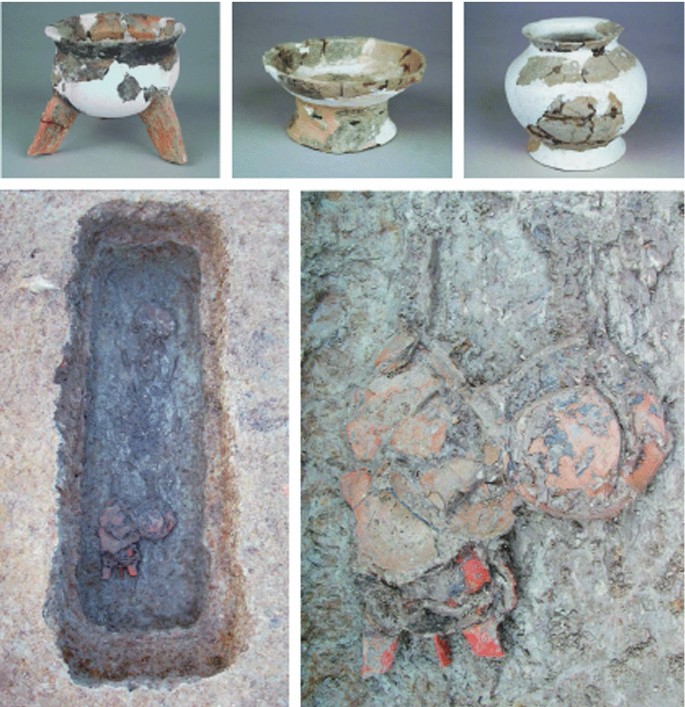The image showcases a collection of archaeological artifacts prominently featuring pottery pieces. At the top, there are three distinct items: the first is a corroded bowl with a white body marred by black and gray chipping, standing on two orange legs; the second is a multicolored dish, in hues of white, green, and pink, with a stand, possibly used as an ashtray; the third is a short, wide, oval-shaped vase that is heavily weathered, primarily white with grayish corrosion. Below these, the bottom left image depicts what appears to be a stone artifact resembling an infant or a tomb, characterized by a long rectangular structure. On the right, there is a less identifiable item comprised of an orange circular shape and an adjacent stone object with red legs, posited to be some sort of tool or armor. All pieces show significant signs of age and wear, indicating they could be ancient relics excavated from a dig site.